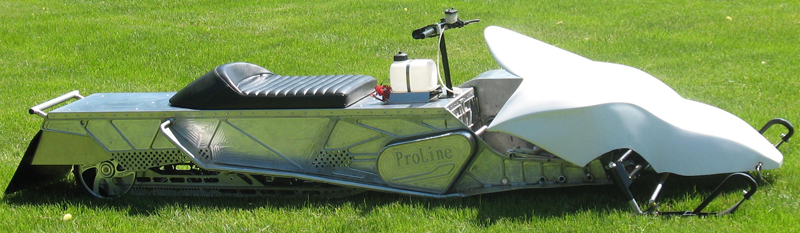The image depicts a unique, long, rectangular machine resembling a snowmobile, placed in a verdant green field under bright daylight. The machine features a sleek, aerodynamic white front shaped somewhat like a stylized dragon or dog head. Its body has a metallic silver chrome hue, complemented by a black seat situated towards the middle. Adjacent to the seat is a white plastic container, likely for gas, and a handle, with lines suggesting connections to brake controls. Stamped directly into the metal below the gas container is the word "ProLine." The machine is equipped with skis at the front and snowmobile-like tracks underneath, supported by a stainless steel cover on the left side. At the rear, part of the machine’s inner workings and the cover for the back wheel are visible. The entire contraption casts a black shadow on the grassy field, emphasizing the clear and bright conditions under which the photo was taken.